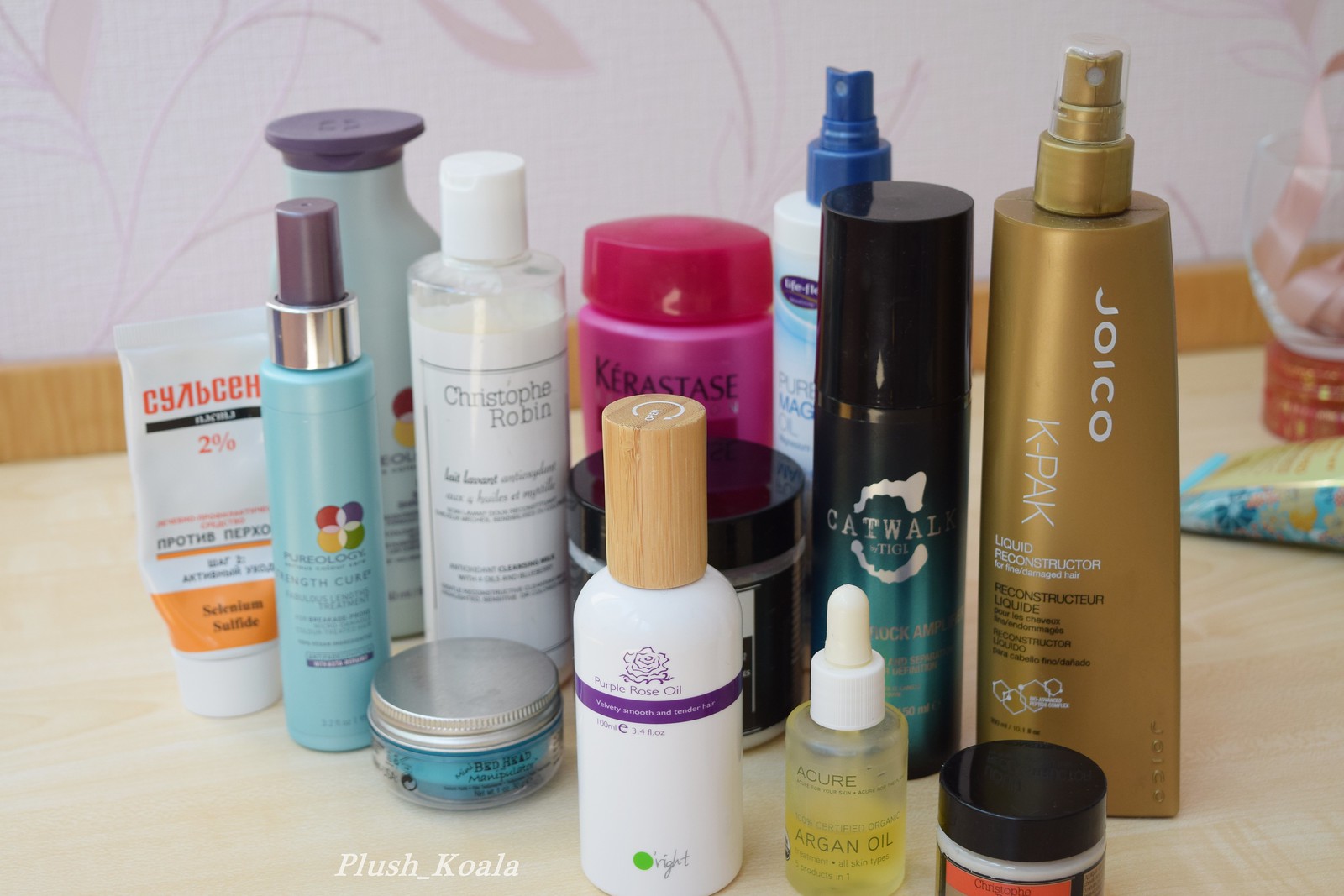A close-up of a bathroom countertop is showcased, adorned with an assortment of beauty and personal care products. The background features white wallpaper adorned with delicate flower motifs, adding a touch of elegance to the scene. Starting from the left, an orange and white squeeze bottle stands prominently next to a vibrant blue spray bottle. Adjacent to this is a sleek white bottle labeled "Christophe Robin," capped with a matching white lid. Flanking this is a stylish pink bottle branded "Kerastase." At the forefront of the image, a transparent glass dropper bottle, filled with Argan oil and topped with a white dropper cap, captures the light, adding a hint of sophistication to the collection. The array of products, ranging from utilitarian squeeze bottles to luxurious dropper bottles, reflects a well-curated selection of daily essentials.